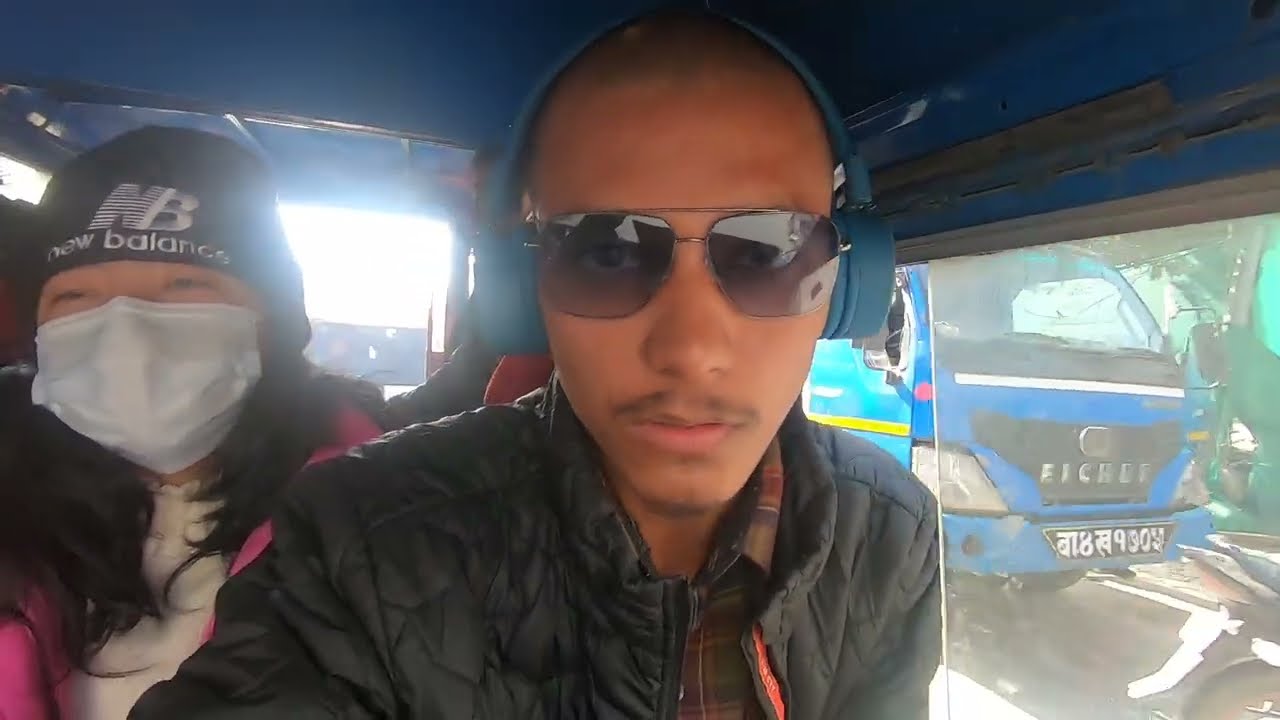The photograph showcases two young individuals, a man and a woman, inside a vehicle, possibly a bus or taxi, situated in what appears to be a foreign country, suggested by the Asian lettering on vehicles outside. The man, positioned centrally and facing the camera, sports very short hair and dons somewhat see-through black sunglasses along with blue over-ear headphones. He is attired in a black jacket, underneath which he wears a collared shirt. A hoodie appears to cover part of his head. To his left, a woman, also looking towards the camera, is wearing a black beanie featuring the New Balance logo and the letters "NB". Her face is partially covered by a white mask, and she wears a pink jacket over a white shirt. Through the window to the man's right, a distinct blue truck is visible with a black grill section that has partially legible lettering starting with "EIC" and a blurred advertisement below reading "8 something 930". The ambiance is bright as light streams through the back window, highlighting the details in this daytime scene.